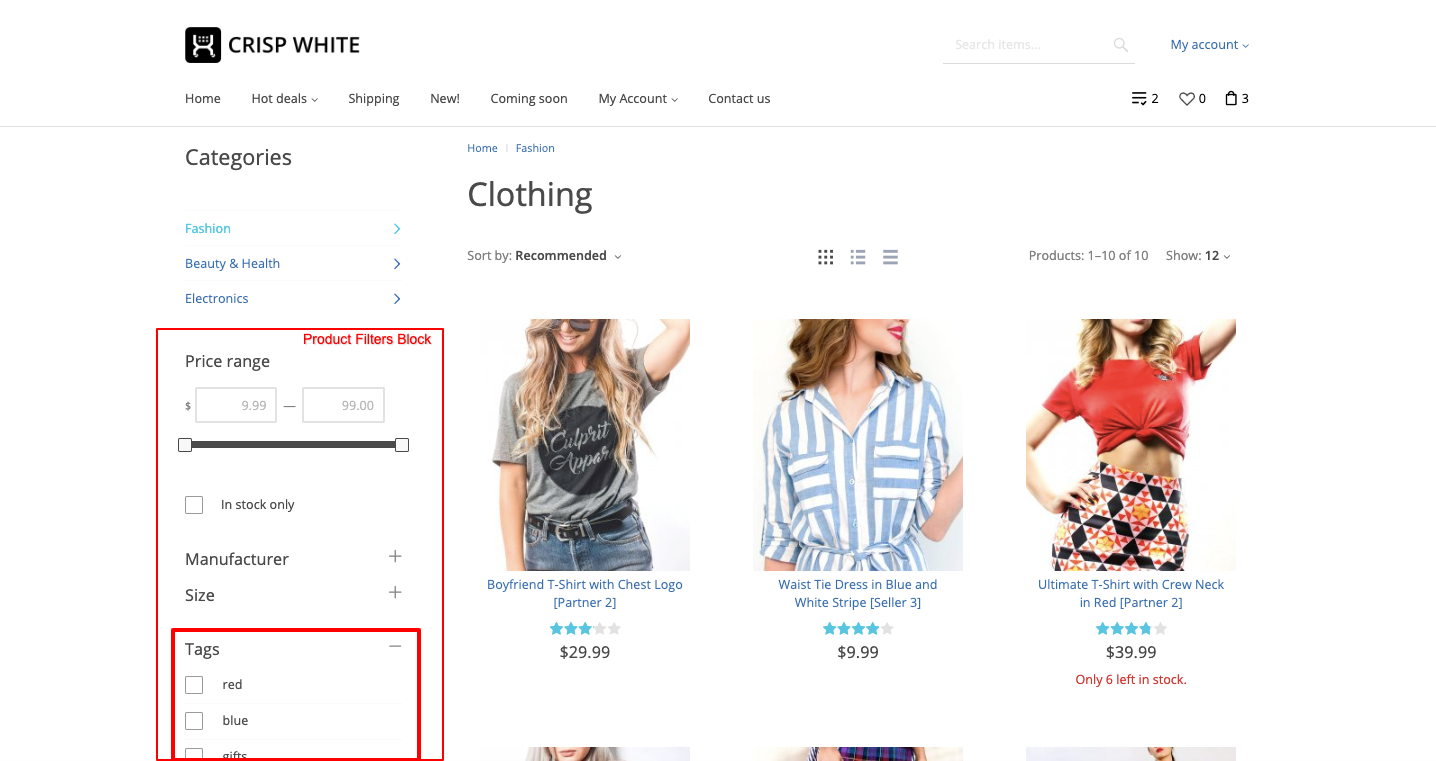This image is a detailed screenshot of a web page titled "Crisp White." At the top of the page, there is a logo within a black box, featuring a stylized 'U' in white, resembling the Under Armour logo. Below the logo, the text "CRISP WHITE" is presented in bold, black capital letters.

The navigation menu beneath the header includes several buttons: "Home," "Hot Deals," "Shipping," "New!" (with an exclamation mark and capital C), "Coming Soon," "My Account" (both words capitalized), and "Contact Us." To the far right of the menu, there are icons in a horizontal row consisting of three vertical lines, a small icon next to it, a heart icon, and a shopping bag icon, which has a cart indicator showing the number '3' in the upper right-hand corner.

On the left side of the page, there is a blue "My Account" button. Just below it, a "Categories" section lists "Fashion," "Beauty and Health," and "Electronics." Following the categories, there is a price range filter with two input boxes and a slider bar, accompanied by an "In Stock Only" checkbox. This price range section is highlighted with a red outline, and there's a red box labeled "Product Filters."

To the right of the filters, the main section of the page displays clothing items. There are product images of a women's t-shirt, a blue and white striped dress with a waist tie, and another t-shirt with a crew neck. Each product listing includes star ratings and the pricing information.